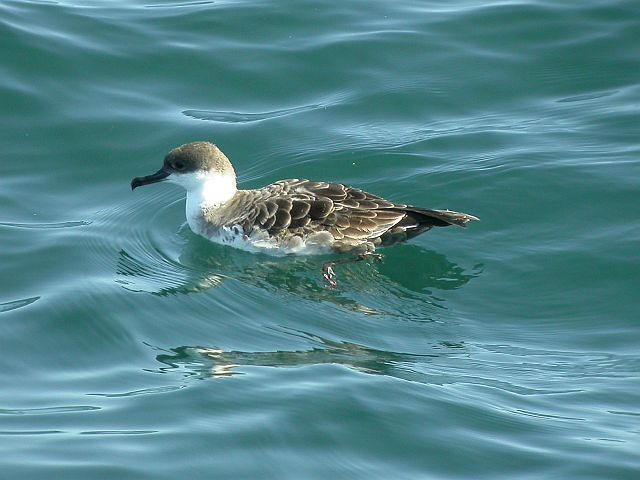The image showcases a close-up of a water bird swimming atop gently wavy, greenish-tinted water. The bird, which resembles a seagull more than a duck, has a distinctive black, pointed beak that curves into a hook at the tip. Its head is primarily light gray with darker gray markings around its eyes, transitioning into a white neck. The bird’s wings and back feature a gradient of gray to darker brown feathers with lighter edges, and its tail feathers are nearly black. The bird's submerged feet create ripples and small waves in the water, which are visible along with some distorted reflections of the bird.